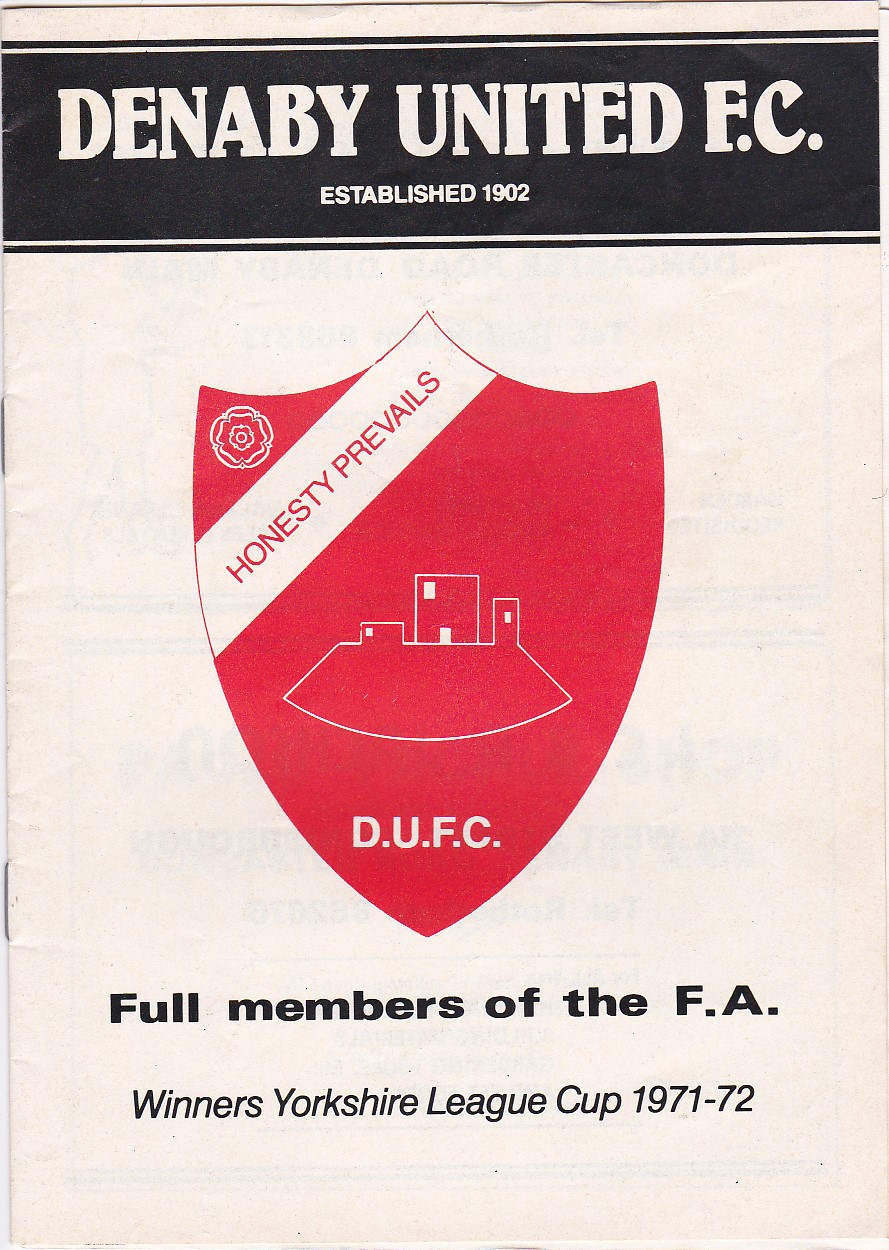The image is the front cover of an old soccer program for Denneby United FC, established in 1902. At the top, a black banner with blue borders holds the club's name written in white font. The majority of the cover is white, with two small staples on the spine. Prominently featured in the center is a red shield or crest containing a white diagonal stripe with the club motto, "Honesty Prevails," written in red text. The crest includes a small flower in the upper left corner and an outline of what appears to be a building on a hill, with the letters "D-U-F-C" below it. Beneath the crest, in black lettering, it states "Full Members of the F-A," followed by "Winners Yorkshire League Cup 1971-72" in italicized font.